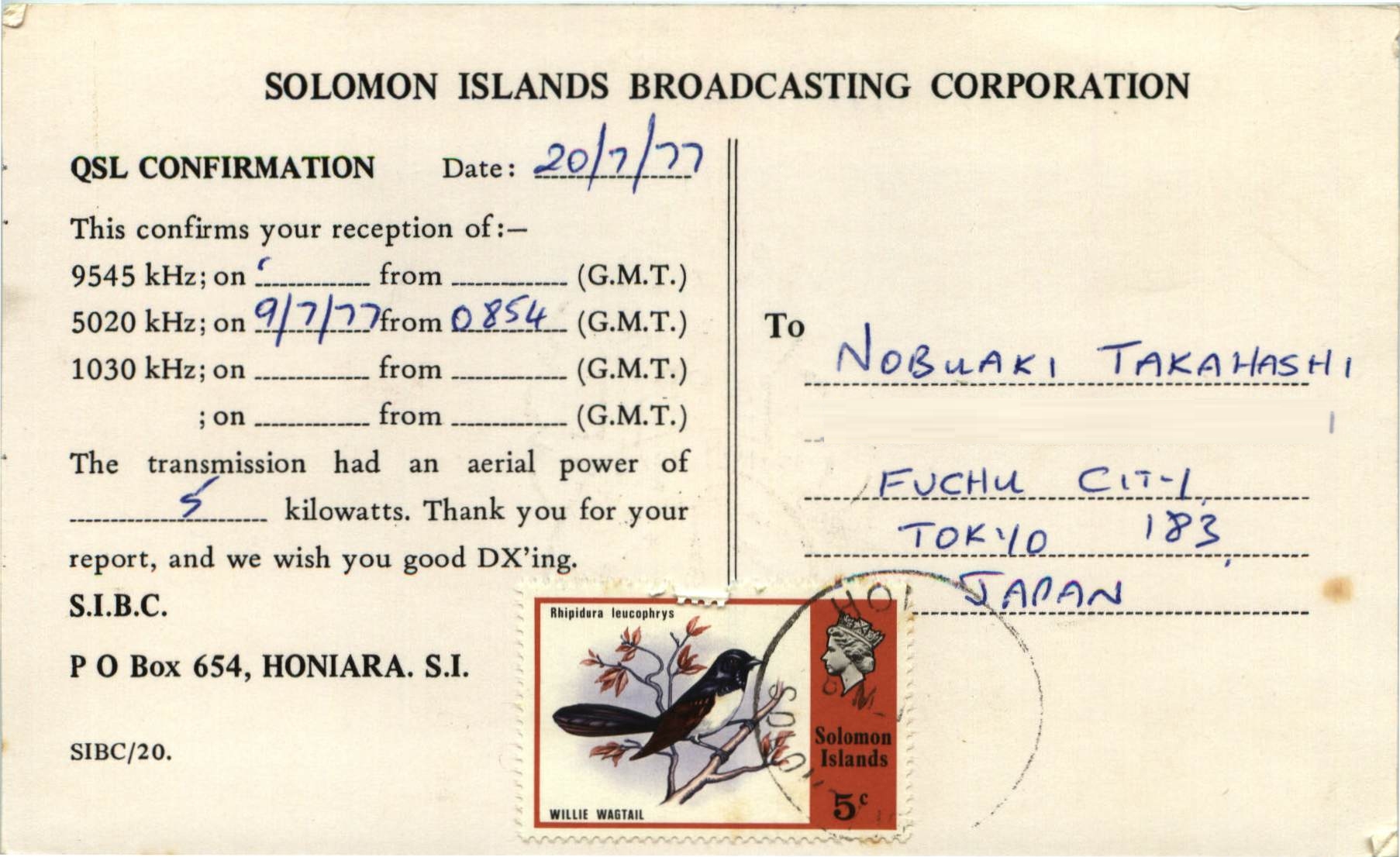This image is a scanned postcard featuring the Solomon Islands Broadcasting Corporation's QSL confirmation. The postcard is off-white beige with visible stains and splotches. Centered at the top, in bold capital letters, it reads "SOLOMON ISLANDS BROADCASTING CORPORATION." Below that, on the left-hand side, it states "QSL Confirmation" with the date "20-7-77." The text confirms the reception of a transmission on "5020 kHz" on "9-7-77" at "0854 GMT." It details the transmission's aerial power as "5 kW" and includes a message: "Thank you for your report. We wish you good DXing." 

The right side of the postcard, beneath two narrow vertical lines, is addressed to "Nobuaki Takahashi, Fuchu City, Tokyo 183, Japan," written in blue pen. A beige and red stamp featuring a black bird roosting on a tree branch with several red leaves and a queen's head face value of "Solomon Islands five cents" is affixed to the card. The return address is "SIBC, P.O. Box 654, Honiara, SI, Solomon Islands," highlighting its origin and corresponding postal details.